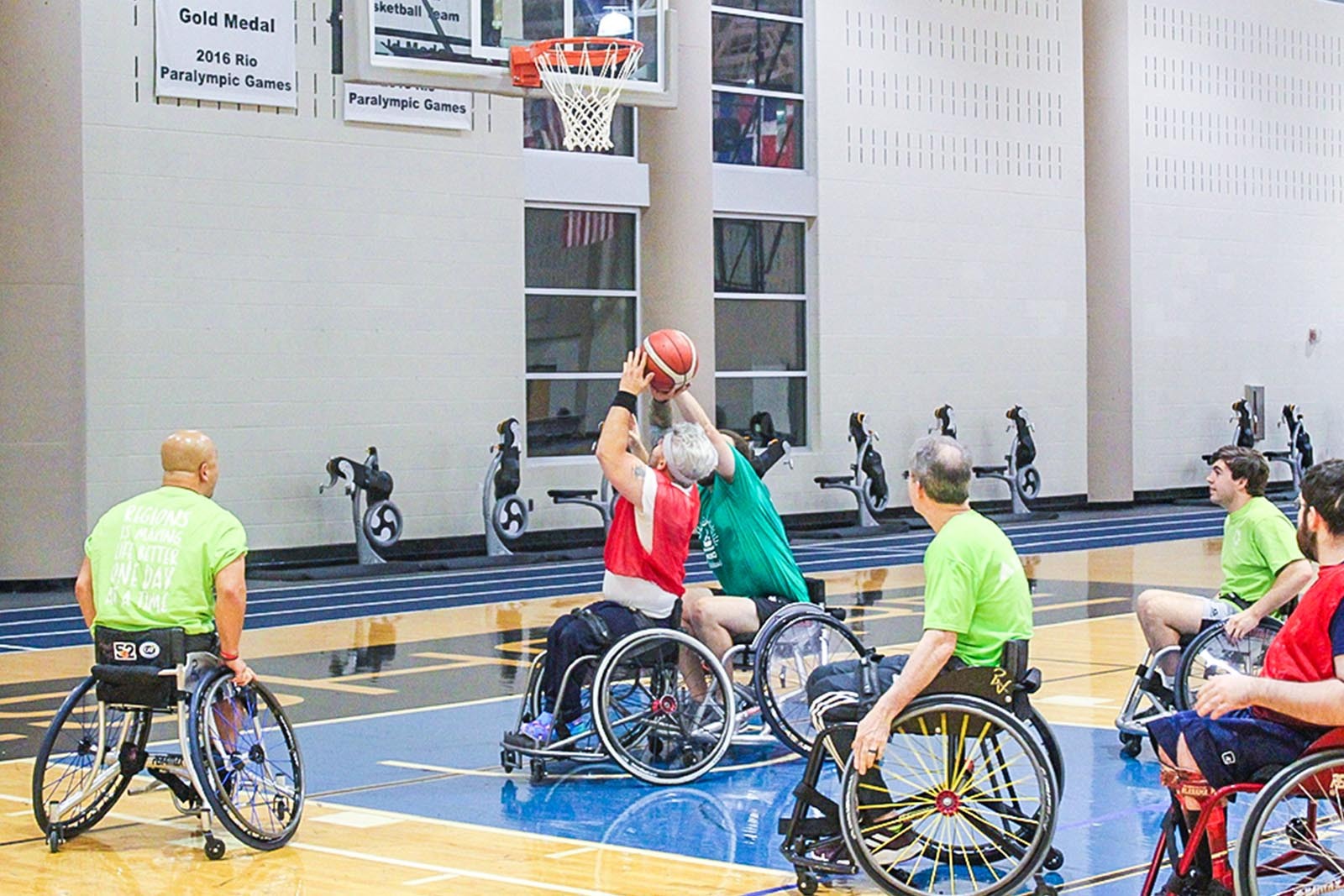In this vivid image, we observe a climactic moment in a thrilling game of wheelchair basketball, set in a brightly lit gymnasium with shiny, wooden floors accented by blue and black paint beneath the basketball hoop. The match features two teams, one dressed in red and the other in varying shades of green, including distinct lime and emerald hues. 

The focal point of the action showcases a player in a red jersey layered over a white t-shirt and blue pants, poised to shoot the ball. A determined opponent in an emerald green shirt and blue shorts is seen blocking the attempt, his outstretched hand almost dislodging the reddish-brown basketball with white stripes. Surrounding them are other players in black, gray, or red wheelchairs, all equipped with the distinctive slanted tires for enhanced agility. 

Various player details include middle-aged and younger men, some bald, others with hair, highlighting the diverse backgrounds of the athletes. Behind them, the gym's walls, made of white-painted brick or cinder block, display banners celebrating significant achievements, notably a "Gold Medal 2016 Rio Paralympic Games" sign. Amid the excitement, exercise equipment like bikes and a blue running track with white stripes can be seen, adding to the dynamic environment of this competitive Paralympic game.